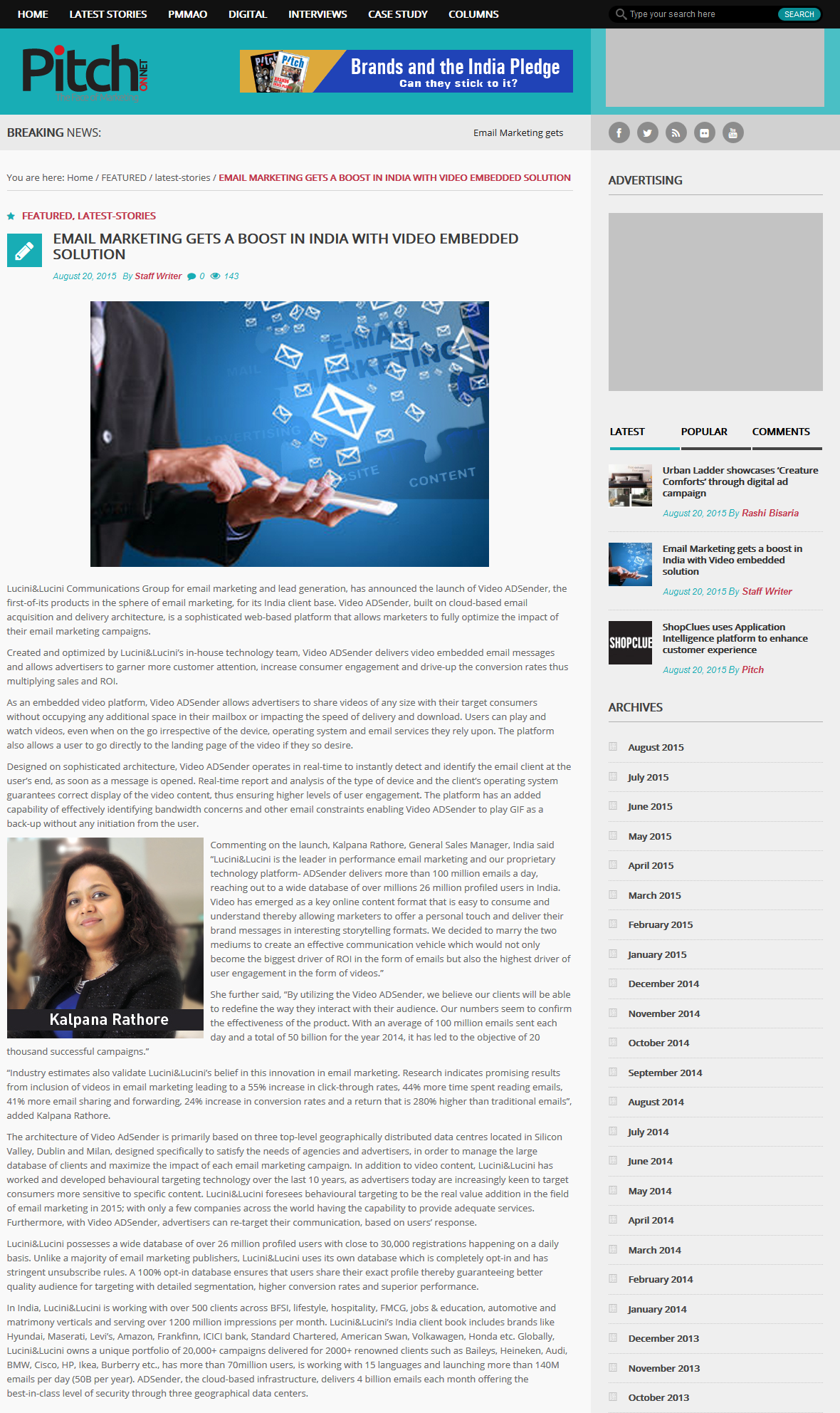This screenshot captures the homepage of the website "Pitch on Net", often referred to as the face of marketing. The top bar of the website features sections in white text against a black background, including Home, Latest Stories, PMMAO, Digital, Interviews, Case Study, and Columns. Beneath this, a header with a blue background displays the Pitch logo on the left and a long horizontal advertisement on the right. The ad highlights that Pitch has two magazine covers with the tagline "Brands and the India Pledge. Can they stick to it?". Adjacent to the advertisement is a search bar in black with a blue search button.

Below this header, the layout includes an empty horizontal gray rectangle labeled "Breaking News" with the headline "Email Marketing Gets...", followed by social media buttons for Facebook, Twitter, Reddit, a message icon, and YouTube. On the right side, an advertising section features another gray rectangle. Directly beneath, links to "Latest", "Popular", and "Comments" articles are presented, with the "Latest" section selected displaying three article titles.

In the center of the screenshot, the "Featured" article section shows the headline "Email Marketing Gets a Boost in India with Video Embed Solution", dated August 20th, 2015, authored by Staff Writer, with 143 views. Accompanying the headline is an image of a man whose face is not visible; only his hands are shown as he uses his phone to send marketing messages. The article itself contains a long, detailed text. To the left, a photo of a woman identified as Kalpana Rathore is also visible.